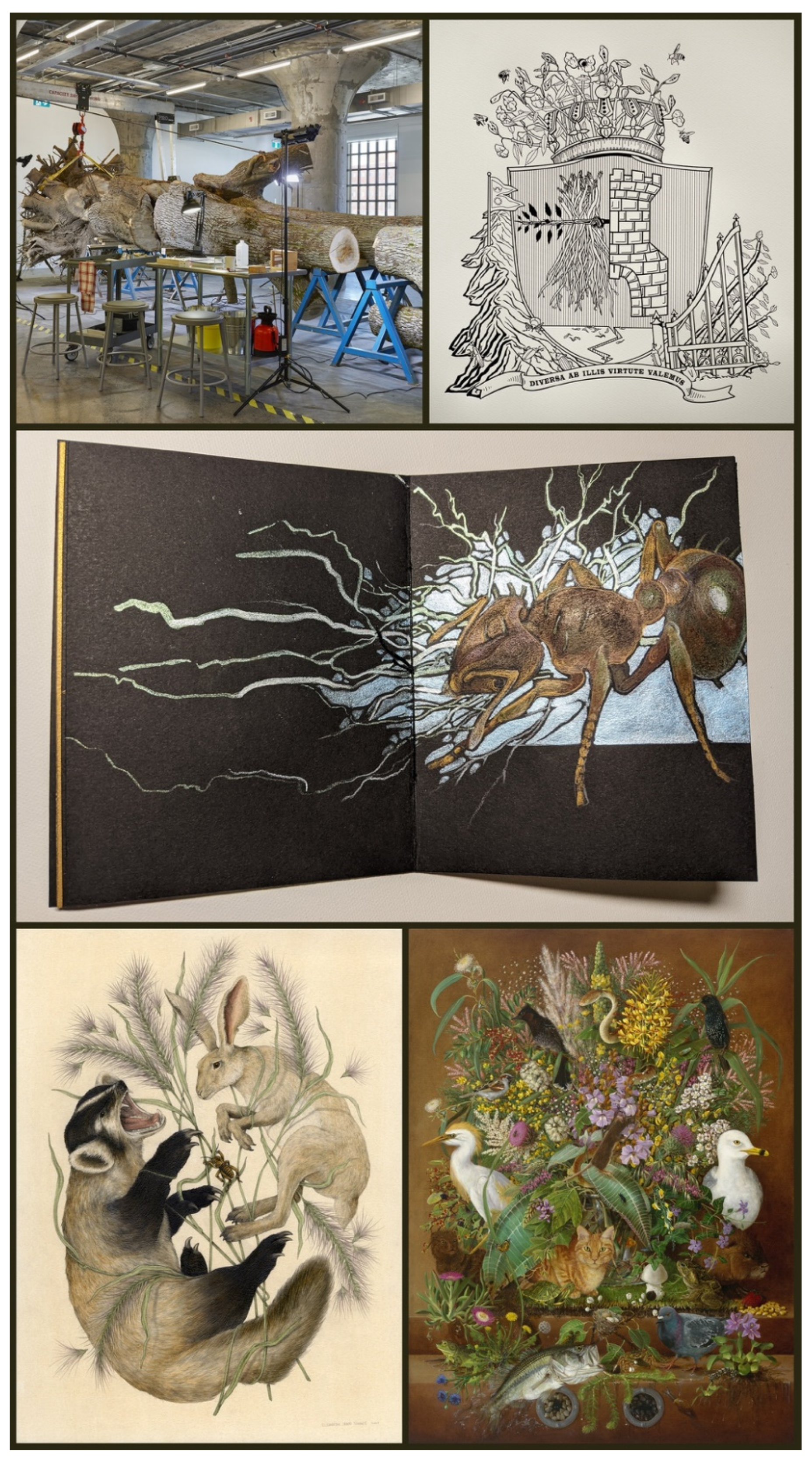This vertical collage consists of five distinct images arranged within a rectangular frame, each separated by a black line. Occupying the upper left cell, there is a realistic photograph of an indoor workshop, featuring a large tree trunk laid across sawhorses and a work table. Surrounding the trunk are various stools and lighting tripods, suggesting an art or woodworking studio setting.

To the right of this image, the upper right cell showcases a black-and-white illustration resembling a coat of arms or crest. The design includes a round circle bordered with detailed florals and possibly the Latin inscription "diversa in illis virtut volimus" at its base.

In the center cell, there is an open book displaying a detailed illustration of a large, brown ant situated against a stark white page. The book itself has a dark brown, worn cover, and the image of the ant contrasts against the white background.

The bottom left cell contains a whimsical drawing of a large hare facing off against a smaller animal, possibly a badger or lemur. Both creatures are surrounded by delicate ferns and other foliage, adding a naturistic charm to the scene.

Lastly, the bottom right cell presents another intricate illustration featuring a lush floral arrangement with pink, purple, and yellow flowers. Interspersed within the flowers are various animals—a prominently placed orange cat, a bird, a fish, and multiple smaller birds—creating a vivid and lively composition.

Together, these images form a diverse vertical montage blending photographic realism and imaginative illustrations.